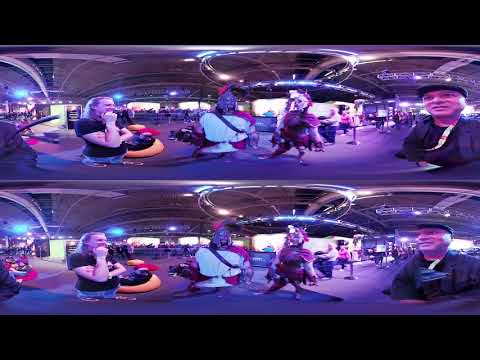This horizontal vertical stereo image, with noticeable lens distortion, captures the vibrant and eclectic scene of an indoor event, possibly at a convention center or Vegas casino, filled with a variety of characters and intriguing elements. Dominating the center of the image are several individuals dressed in elaborate Roman cosplay attire, reminiscent of ancient Spartans. On the right side, a man in a newsboy cap is prominently situated, adding a touch of historical charm. To the left, an individual clad in denim shorts and a black t-shirt stands contemplatively with their arms crossed and chin resting on their right fist, gazing at the Roman cosplayers with curiosity.

The image appears to be a composite of two nearly identical photos stacked vertically, creating a slightly distorted, surreal effect reminiscent of a 360-degree camera demonstration. The background showcases a spacious venue with visible metal girders and infrastructure, further emphasizing the indoor setting. The lighting casts a purple hue across the scene, adding to the distinctive and slightly whimsical atmosphere. Despite the unusual combination of elements, the people in the image remain unfazed, suggesting that such vibrant and diverse displays are a common sight at this event. The color palette includes shades of black, purple, yellow, orange, red, white, blue, and gray, enhancing the dynamic and colorful ambiance of the moment.